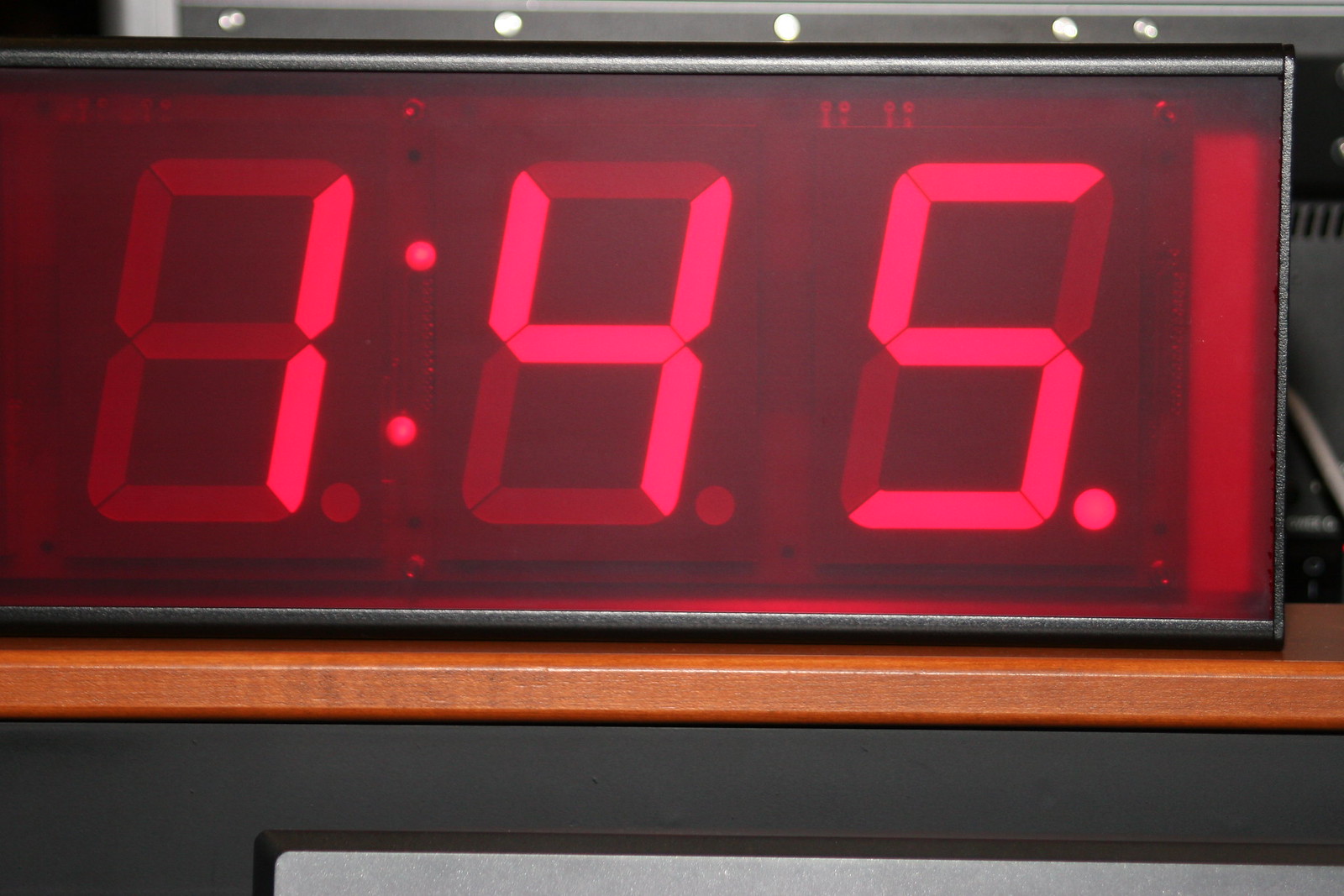The image depicts a close-up view of a digital clock or timer. The device, encased in a simple black metal or possibly silverish frame, prominently displays the time "1:45" in bright red digits. The clock face, with a dark red or black background, also faintly reveals the full outlines of all potential digits, forming an "888" pattern when not lit. The clock is positioned on a thin wooden shelf, beneath which a black section is visible. In the lower right corner, a small silver square protrudes slightly. Behind the clock, some electronic equipment and a gray beam can be discerned, adding context to the setting. The close-up nature of the photograph emphasizes the details and construction of the timekeeping device.